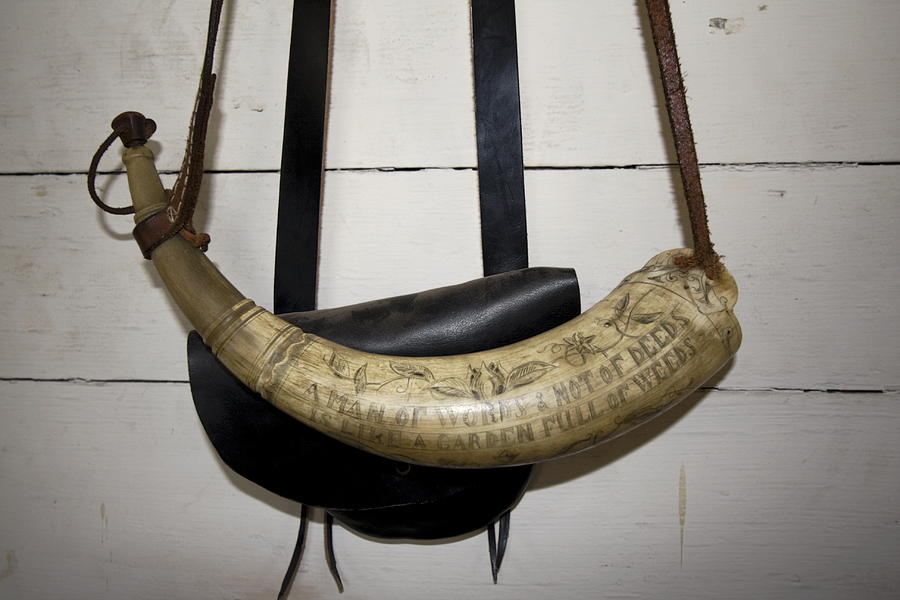The photograph features a detailed and rustic scene on a white-painted, weathered wooden wall, likely outdoors given the visible gouges and marks on the paint. Mounted on this wall is a black leather satchel, positioned from the top middle down towards the lower middle, distinguished by its half-moon shape and two thick leather straps. The satchel also features a button closure and four strings, two descending from each side.

Hanging prominently in front of the satchel is an intricately crafted drinking horn, possibly made from a sheep's or bull's horn. The horn boasts polished, shiny ivory-colored exterior with scrimshaw engravings, including a silhouette of plants, flowers, and leaves. The centerpiece of the engraving displays the aphorism: "A man of words and not of deeds is like a garden full of weeds." This horn, designed with practicality in mind, features a dark brown leather plug at its narrow end and is suspended by brown leather straps attached at both ends. The meticulous craftsmanship and the rustic charm of the setting create a vivid and poignant tableau.